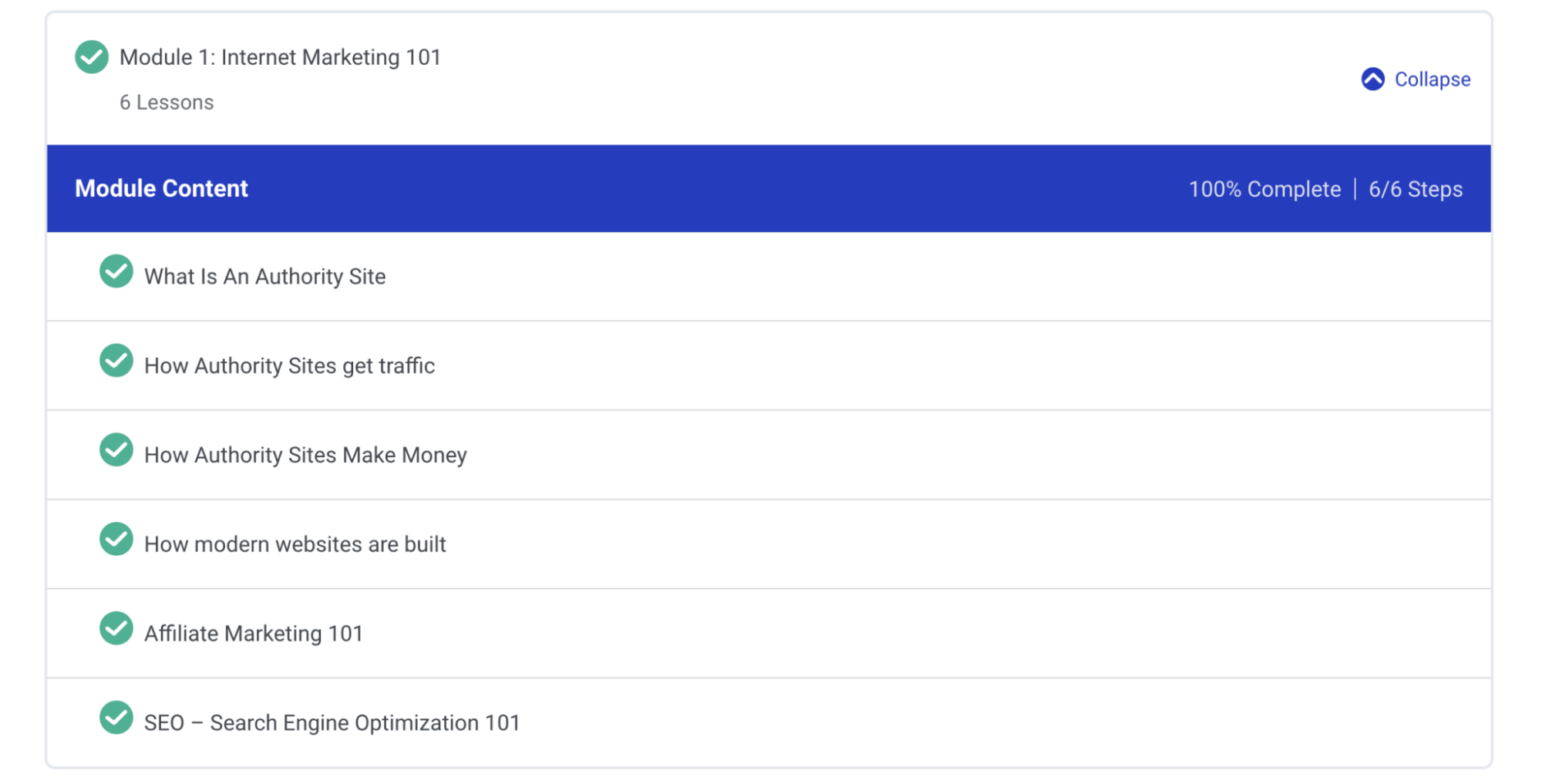Screenshot Description:
The image captures a webpage titled "Internet Marketing 101," displayed as Module 1 of an online course. The heading "Module 1, Internet Marketing 101" is prominently featured at the top, followed by a list of six lessons, each marked as complete. To the left of the module title is a green circle containing a white checkmark, indicating the module's completion.

On the upper right-hand side of the module title, there is a collapse icon that allows users to expand or collapse the module content. Below the title, a long rectangular blue bar reads "Module Content, 100% Complete, 6/6 steps," signifying that all lessons within the module have been completed.

The six lessons listed under the module are:
1. What is an Authority Site?
2. How Authority Sites Get Traffic
3. How Authority Sites Make Money
4. How Modern Websites Are Built
5. Affiliate Marketing 101
6. SEO - Search Engine Optimization 101

Each lesson is presented as a separate line item, enclosed in its own box. To the left of each lesson title is a green circle with a white checkmark, denoting the completion status of each. The entire screenshot is framed by a blue border, creating a cohesive and structured appearance.